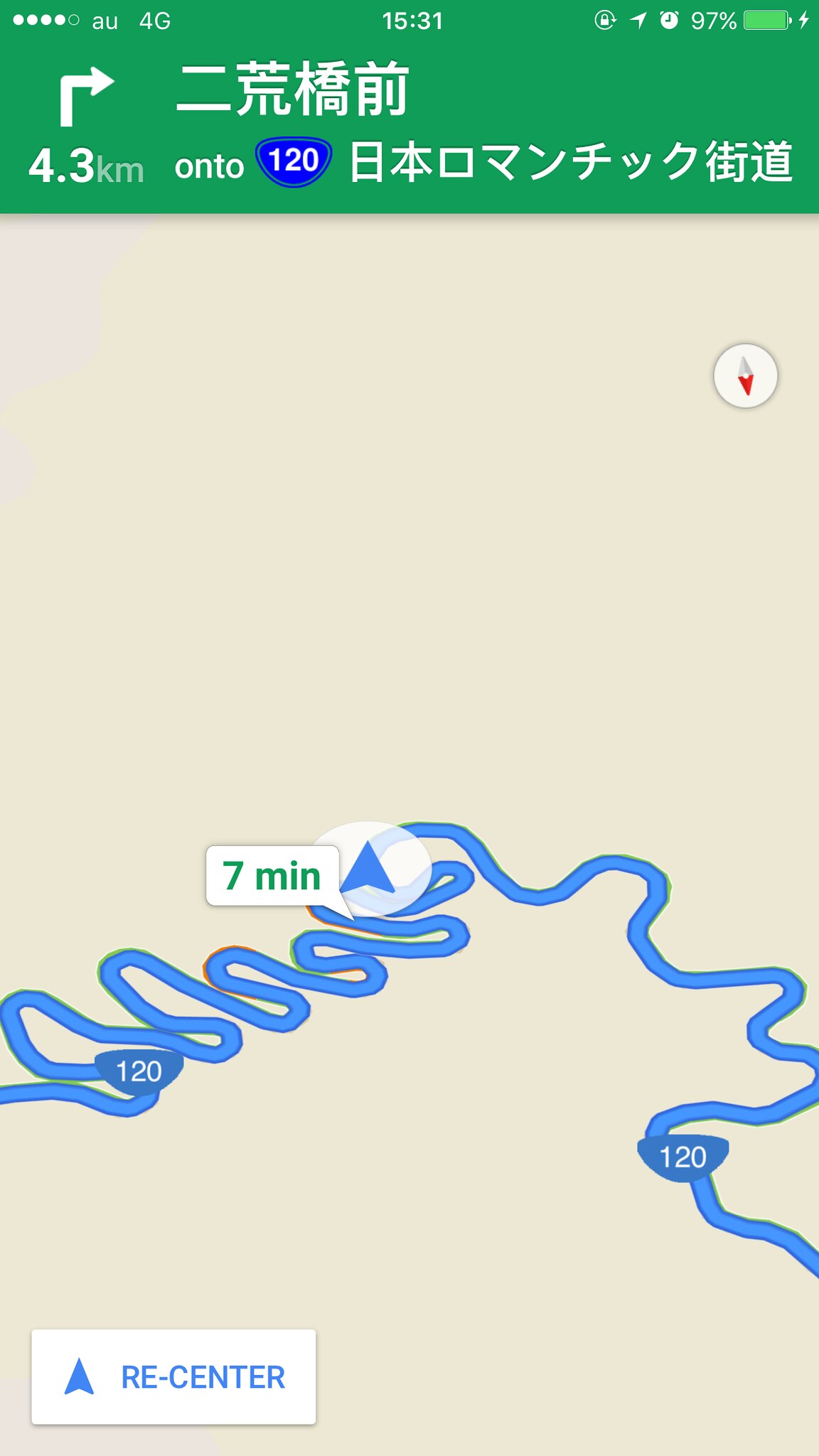This screenshot from a phone screen captures the navigation interface of a map application, possibly Google Maps. At the top, a green status bar displays various icons: on the left, five dots with four filled in white and one outlined, indicating signal strength; in the middle, the time reads "15:31"; and on the right, several icons indicate current settings - a location icon, an alarm set, a battery percentage of 97%, and a lightning bolt symbol for charging.

Beneath the status bar is text in a foreign language, possibly Chinese, Japanese, or Korean. Following this text, it indicates a distance of "4.3 kilometers" and a reference to "120," again with more foreign characters.

Dominating approximately 80-90% of the screen is a khaki-colored map section showcasing a zoomed-in route. In the top-right corner of this section, there is a small compass icon. The route itself is depicted as a very squiggly and winding blue line with a darker blue outline, resembling a meandering river. A blue arrow encircled by a white border marks the current location, accompanied by a label indicating "seven minutes." 

In the bottom-left corner, a rectangular button featuring a location symbol and blue text that reads "re-center" provides an option to re-center the map to the current location. This detailed screenshot encapsulates various elements of navigation while on the move, providing a comprehensive view for the user.